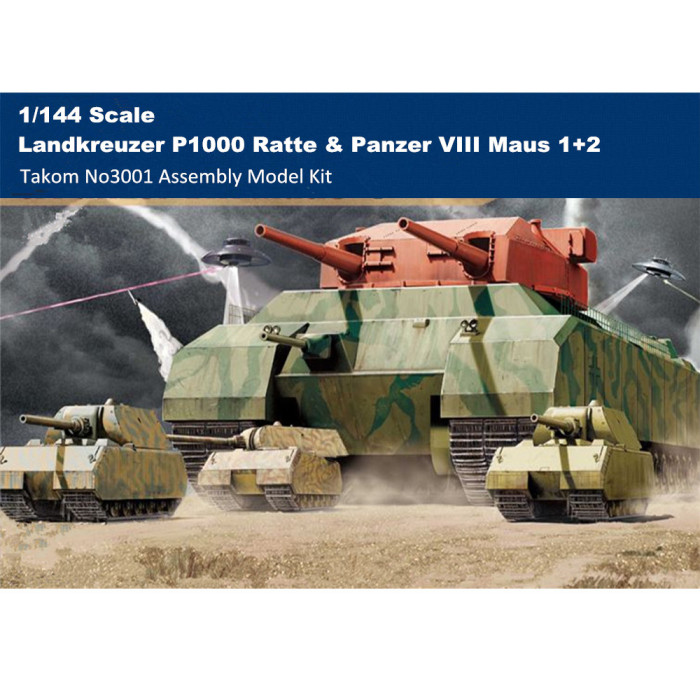The image showcases an advertisement for a model kit of military tanks. At the top, a navy blue header spans the width of the image with white text reading, "1-144th scale Landkreuzer P1000 RAT and Panzer VIII Maus 1 plus 2, TACOM number 3001 assembly model kit." Below this header, a detailed scene unfolds featuring a giant military tank painted in dark green and olive camouflage with a distinct red rotating turret equipped with two bright red cannons. In front of this massive tank are three smaller tanks: one with beige and green camouflage, one with beige and brown stripes, and one in solid olive green.

These tanks are depicted moving across a painted brown dirt surface, navigating a desert-like area. The background is dominated by a deep grey, cloudy sky. Adding a touch of science fiction, two flying saucers hover in the sky on either side of the large tank, each emitting white cone-like beams. The saucer on the left is firing a noticeable pink laser beam downward, adding to the dramatic atmosphere of the scene.